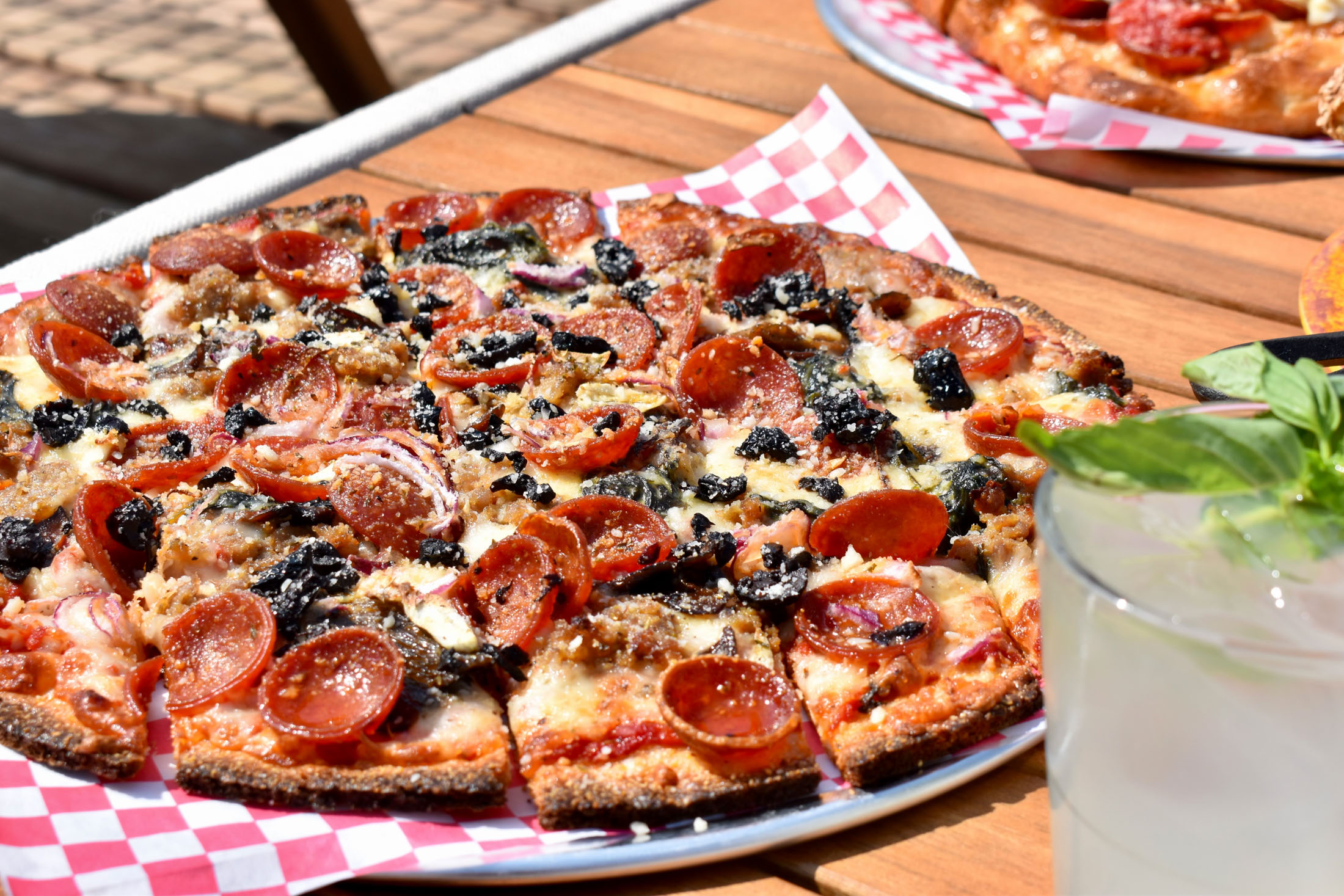On a bright, sunny day, a delectable thin-crust pepperoni pizza is prominently displayed on a wooden table with metal edges, creating an inviting al fresco dining scene. The pizza, resting on a metal tray lined with red and white checkerboard wax paper, is adorned with generous toppings of pepperoni, black olives, and an enticing blend of white and golden brown melted cheese. Nearby, a refreshing glass of lemonade garnished with mint leaves sits filled to the brim, adding a refreshing element to the setting. The outdoor patio atmosphere is captured with sunlight casting shadows, highlighting the vibrant and inviting presentation. An additional piece of pizza and a blurred plate in the background hint at the shared meal that is about to be enjoyed, completing this picturesque and mouthwatering scene.